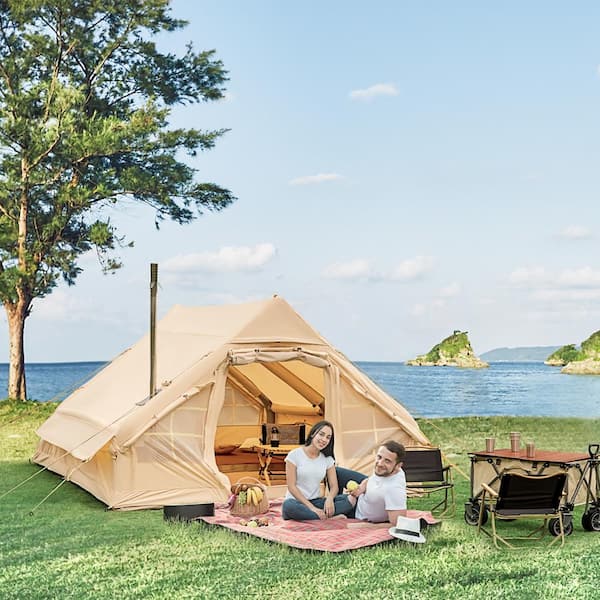The image depicts a young couple enjoying a tranquil outdoor setting on a grassy lawn beside a large body of blue water, reminiscent of both an ocean and a lake. The sky above is a bright blue with some clouds scattered across. The couple is sitting on a picnic blanket that is red and plaid, in front of an advanced, tan canvas tent with low sidewalls and a peaked roof. The tent, pitched on the green grass, features a wooden frame inside and has a metal chimney protruding from its left side, suggesting a heater. Inside the tent, there is a bed and a small table.

To the left of the tent, there is a tree and an area of grass, enhancing the nature-inspired ambiance. The couple, both dressed in white shirts, with the woman also wearing blue jeans and having black hair, are positioned comfortably — the man lying on his side and the woman sitting cross-legged. A basket filled with fruit, including bananas, is placed on the blanket. A table made from a wagon along with two black and yellow folding camping chairs are also set up nearby. To the right of the scene, a fabric or canvas wagon resembling a stroller is visible. The background showcases serene blue water, dotted with several islands and large rocks adorned with green grass or weeds, providing a picturesque contrast to the meticulously arranged camping setup.